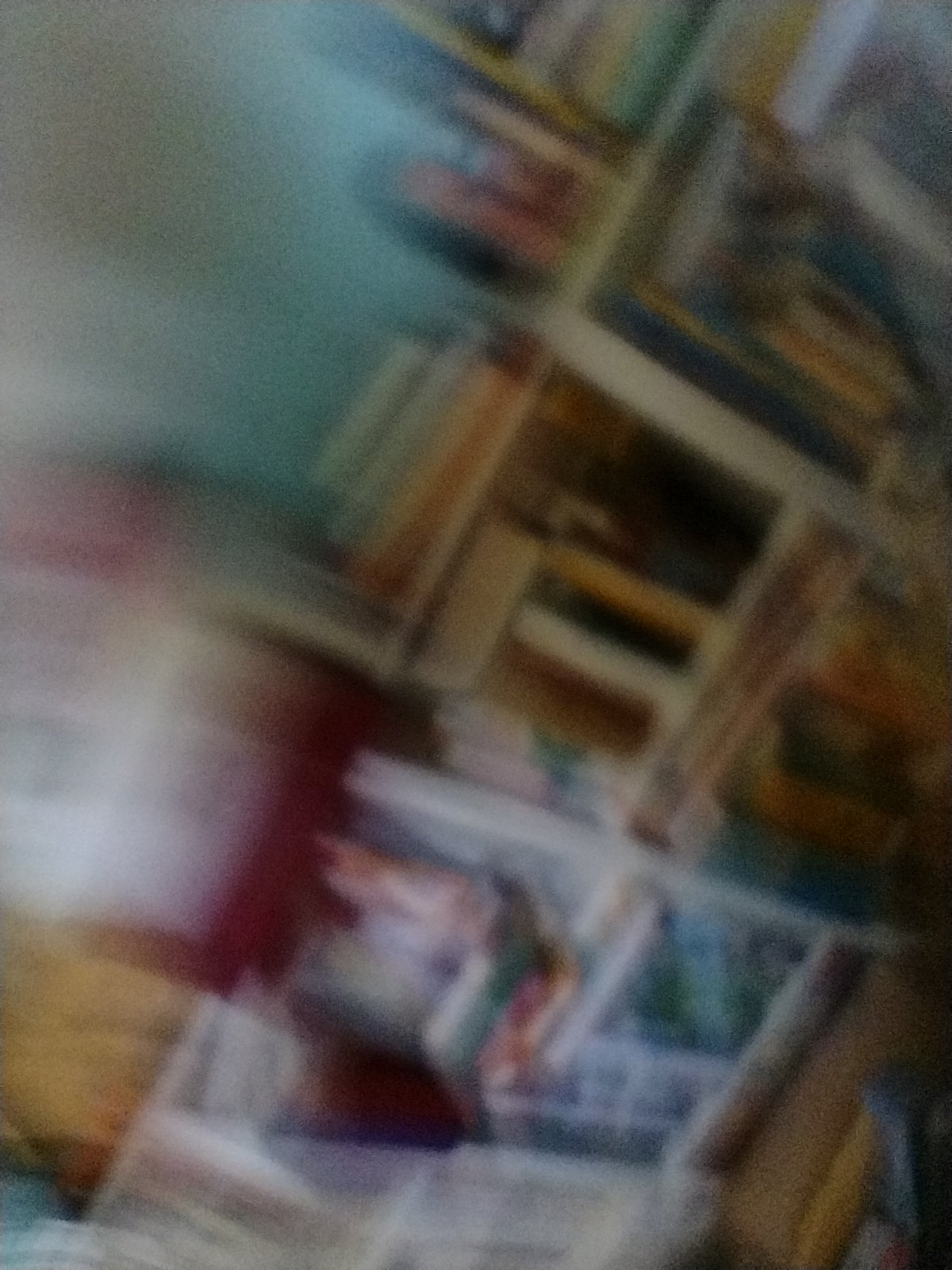The image showcases a white background adorned with an array of items, likely greeting cards or similar types of cards, arranged sophisticatedly on shelves that resemble those found in a library. The shelves' contents reveal a variety of book bindings in shades of white, yellow, and white wood. At the top of these shelves are several more books stacked horizontally. On the bottom left, a series of bordered images or pictures stands out with white framing, while the very bottom of the image has a wooden surface. Scattered throughout the shelves are numerous folders, adding to the organized yet eclectic visual feel. The top-right and top-left corners of the image are slightly fuzzy, with visible patches of light. A red wall and a yellow curtain add a splash of color to the scene, complemented by additional hues such as red, yellow, and green dispersed throughout the composition.